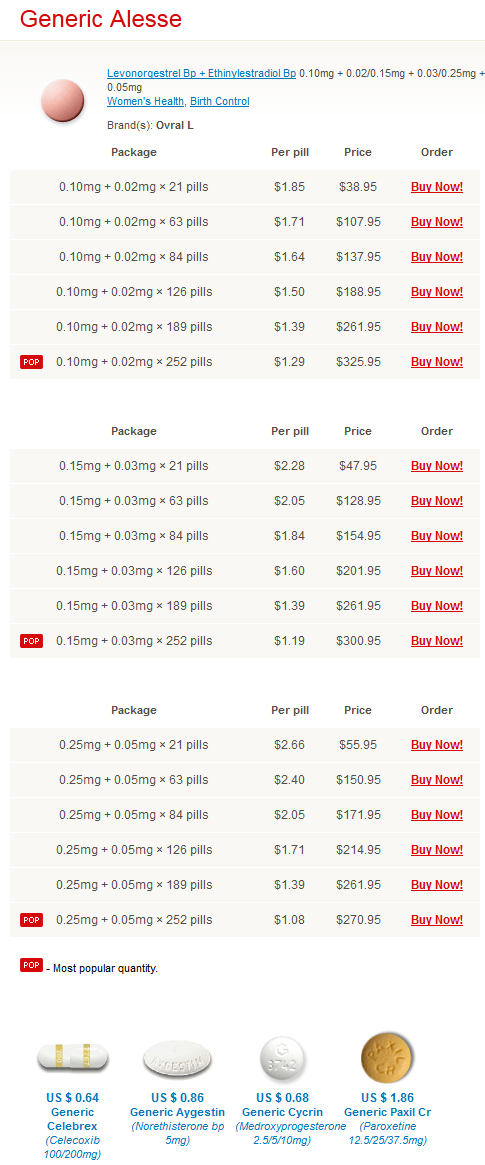This image showcases a section of a website dedicated to women's health and birth control options. At the top left corner, there's a brown pill prominently displayed. The website's header features long names written in blue, indicating various contraceptive options. Directly beneath this header, in blue text, it reads "Women's Health Birth Control."

The content details various birth control pills, categorized by dosage and quantity. The price per pill ranges from $1.29 to $1.95, and the total price is calculated accordingly. Each category includes a red "Buy Now" button for easy ordering. There are package deals available, with the price per pill slightly reduced in some instances, ranging from $1.19 to $2.20, again accompanied by "Buy Now" buttons in red.

Further down, the image highlights the "Most Popular Quantity" section, featuring four different types of pills: an oval-shaped pill with two yellow stripes, an oval white pill, a round white pill, and a round brown pill. All pills are identified as generic with prices varying from $0.64 to $1.86 for the brown pill.

The layout is user-friendly, allowing for a straightforward selection of the desired birth control option, dosage, and quantity.